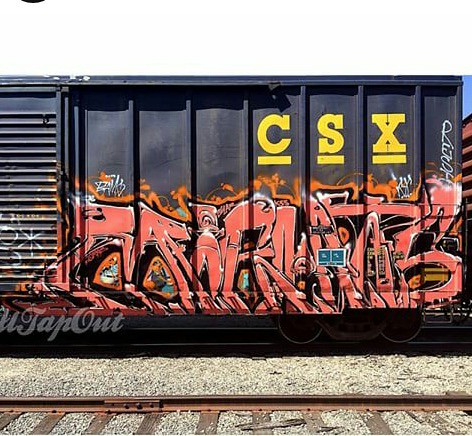In this outdoor photograph of a train yard, a black cargo train car is prominently featured. The train car bears the yellow, underlined letters "CSX" at the top. The lower portion of the train is adorned with intricate graffiti, incorporating various colors such as peach, pink, light red, and designs in orange and white. Some of the graffiti resembles artistic text, including the phrase "tap out" among other unreadable words and symbols. Surrounding the train car, the scene displays a railway landscape with railroad ties, rails, and gravel, along with an adjacent empty track.